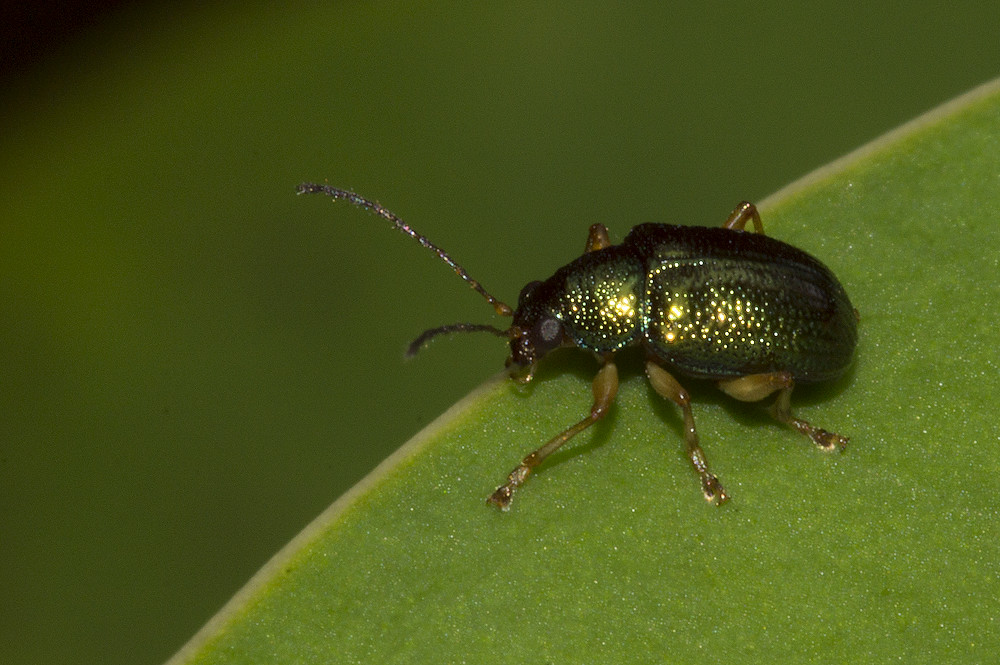This image features a striking, unusual beetle with a metallic green body adorned with light yellow speckles and some black markings. The beetle, which is positioned on a light green, yellowish leaf, showcases its six legs that are a lighter shade of green compared to its body. Prominently visible are its two long antennae extending from the front of its head. One of its gray eyes is discernible, as are its small, front pinchers, seemingly poised to feed on the leaf. The background on the left side of the image fades into a blurred green, keeping the beetle and its vibrant habitat as the focal points.